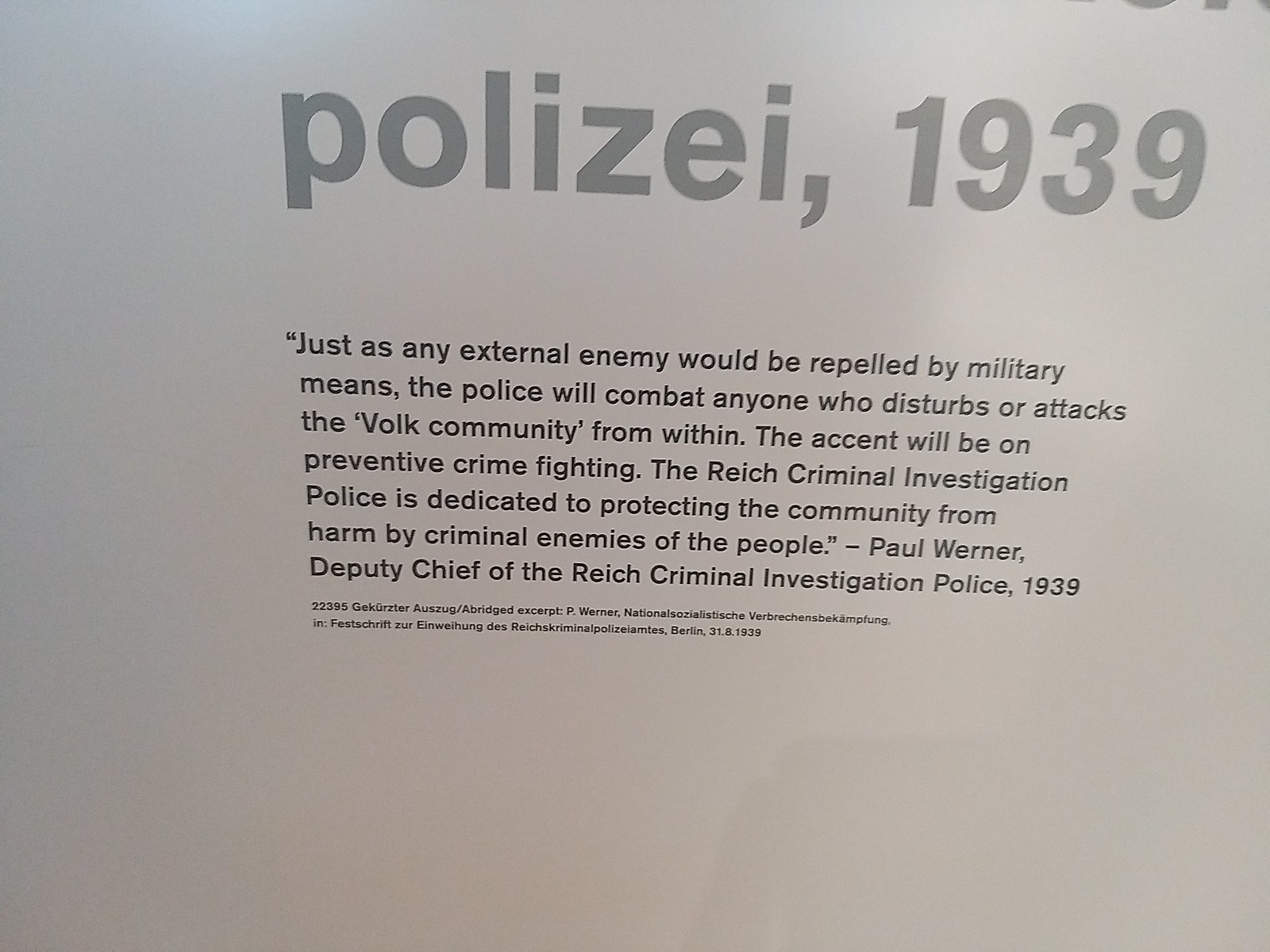The image captures a rectangular white poster board displaying a bold heading at the top that reads "Polizei, 1939" in large gray letters. Below this, a paragraph in smaller black font states: "Just as any external enemy would be repelled by military means, the police will combat anyone who disturbs or attacks the Volk community from within. The accent will be on preventative crime fighting. The Reich Criminal Investigation Police is dedicated to protecting the community from harm by criminal enemies of the people." This quoted statement is attributed to Paul Werner, Deputy Chief of the Reich Criminal Investigation Police, 1939. Additionally, there are some faint, hard-to-read German words along with "Berlin" in black and white, located beneath the main paragraph.